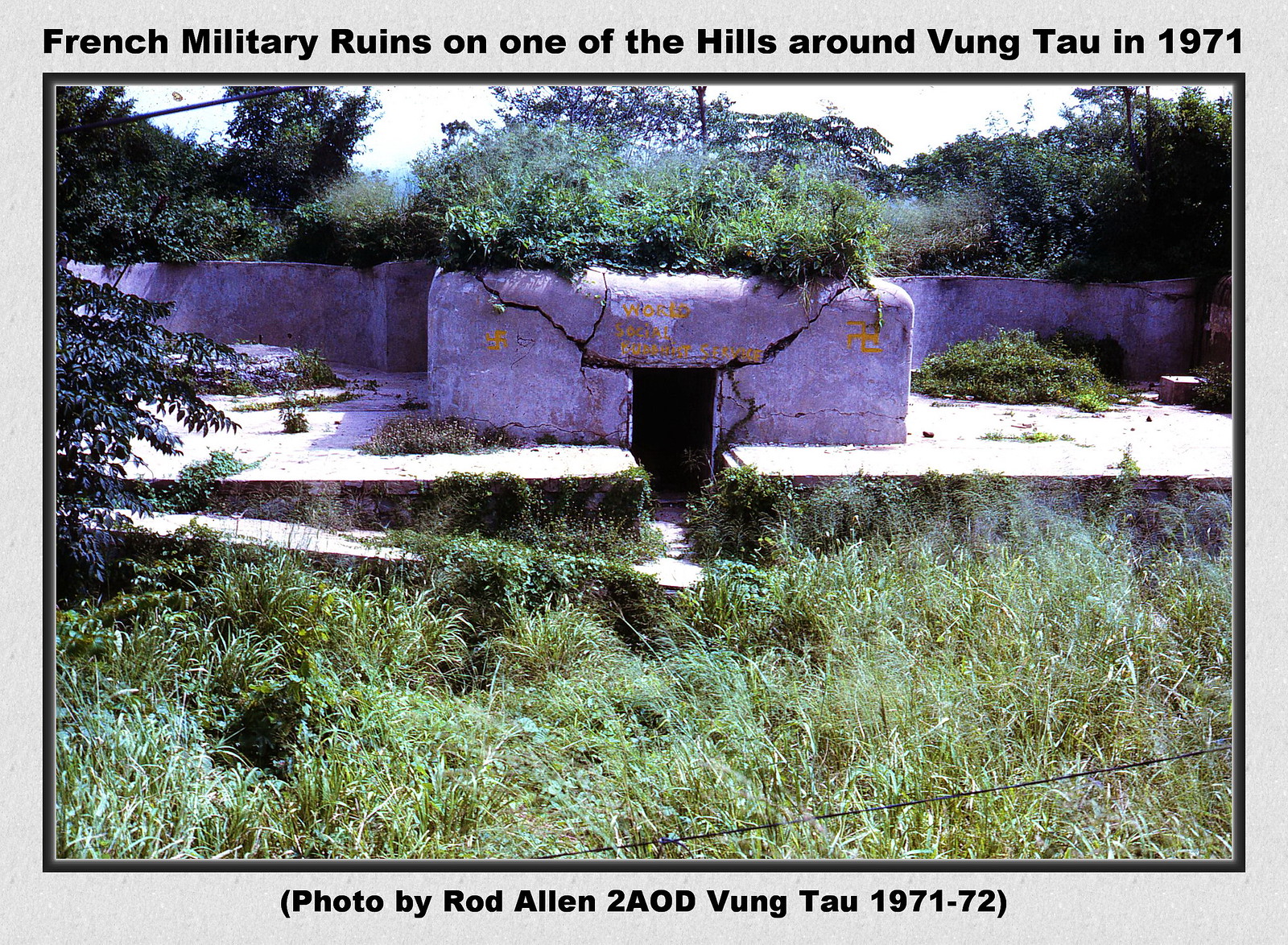The photograph, likely featured in a vintage issue of National Geographic, is enclosed in a black-bordered text box. The caption above the image reads, "French Military Ruins on one of the hills around Vung Tau in 1971," while the credit below states, "Photo by Rod Allen, 2A OD, Vung Tau, 1971-1972." The picture captures an evocative scene of overgrown grasses and weeds enveloping a stark, white concrete bunker standing as a relic of the Vietnam War era. The cracked and weathered structure, marked with yellow inscriptions, has an entrance leading to a dark, possibly hidden interior. Flanked by trees on the left and back, the bunker is subtly embedded in a landscape of tall grasses, with a low surrounding wall crossing from left to right near the top of the frame.